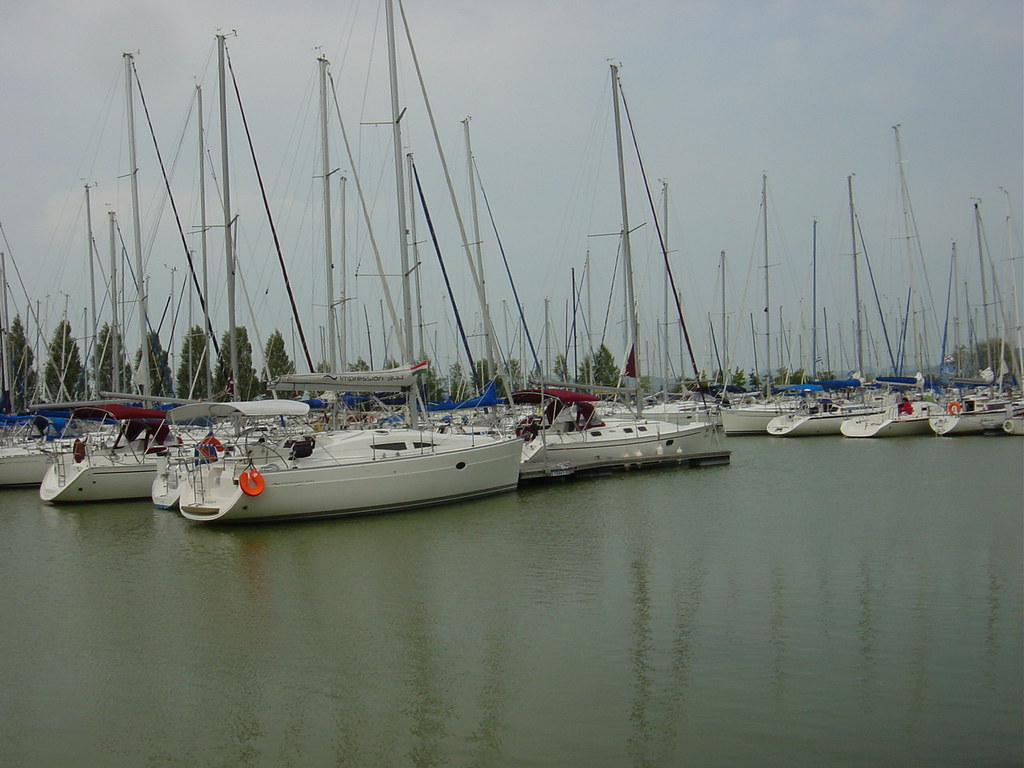This color photo features a muted and overcast marina scene. The water, appearing as a gray-green or brownish moss green, is calm with slight ripples and a bit of reflection. Numerous white sailboats without sails are neatly docked in double rows along multiple docks, their masts extending into the gray sky. The foreground prominently displays several boats; one has an orange life ring visible, and a couple may even have faint figures aboard. Rows of sailboats extend into the distance, with blue and maroon awnings among the white bases. Behind the boats, a planted line of evenly spaced pine trees forms the horizon under the overcast sky.